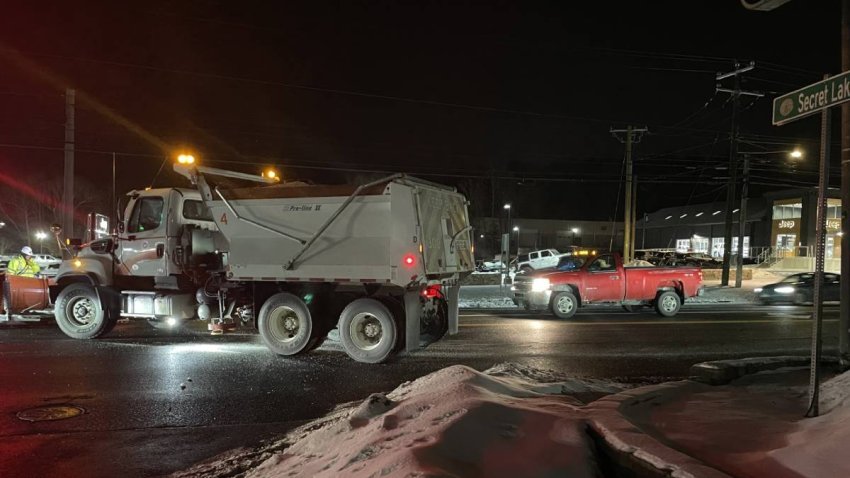In this nighttime winter scene, a bustling city street is captured in the midst of ongoing snowplow work. Snow is piled up along the curb, and an orange plow attached to a large grey dump truck dominates the left lane, recognizable as a salt truck. Accompanied by a worker in a neon yellow jacket with reflective strips and a white hard hat, the scene is set against the backdrop of a one-story building and a Jeep dealership. Traffic continues to flow with a red pickup truck in the right lane and a black sedan in the far lane, both with their headlights piercing the night. Street lights and power lines cut through the darkness, illuminating a road sign partially visible on the curb reading "Secret Lake." Amidst the construction activity, another worker in high-visibility gear is also seen, adding to the detailed portrayal of winter urban life.